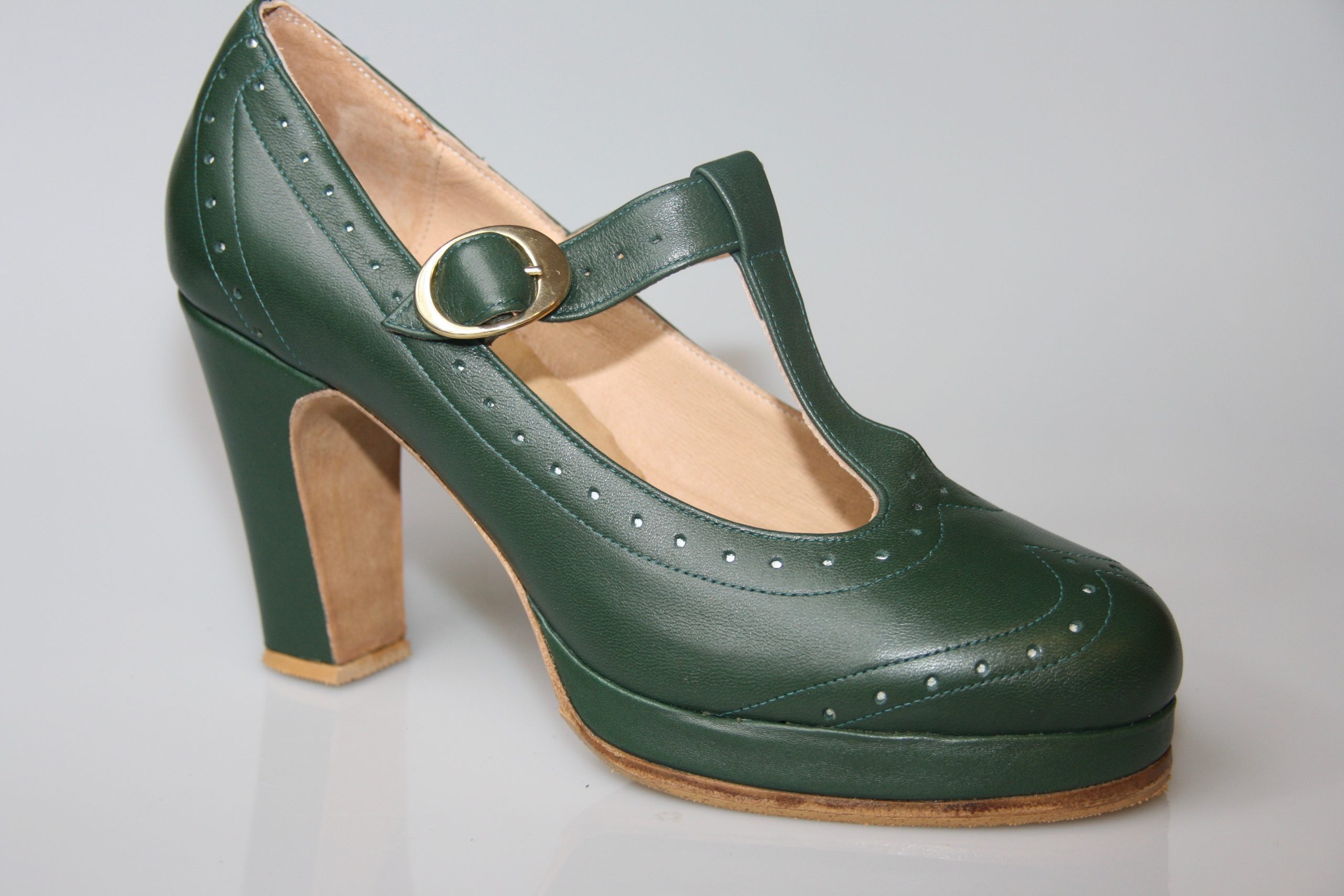This photograph features a detailed side view of an elegant, old-fashioned women’s high-heeled shoe with a distinct combination of colors and intricate design elements. The shoe, crafted from dark green leather, showcases a unique blend of fashion styles; its overall structure resembles that of a classic pump with a boot-like front toe cap. The toe cap is adorned with white perforated stitching that forms a triangular pattern, adding a sophisticated touch. The insole is tan or light brown, matching the outsole and the base of the heel. The heel itself, which has a square-shaped base, is supported by a light brown section that seamlessly blends with the rest of the sole. 

A strap runs over the top of the shoe, securing with a golden buckle, providing both functional support and an elegant accent. The shoe rests on a plain, light gray surface, which contrasts subtly with its rich, dark green and brown hues, highlighting the intricate details and craftsmanship of the shoe.